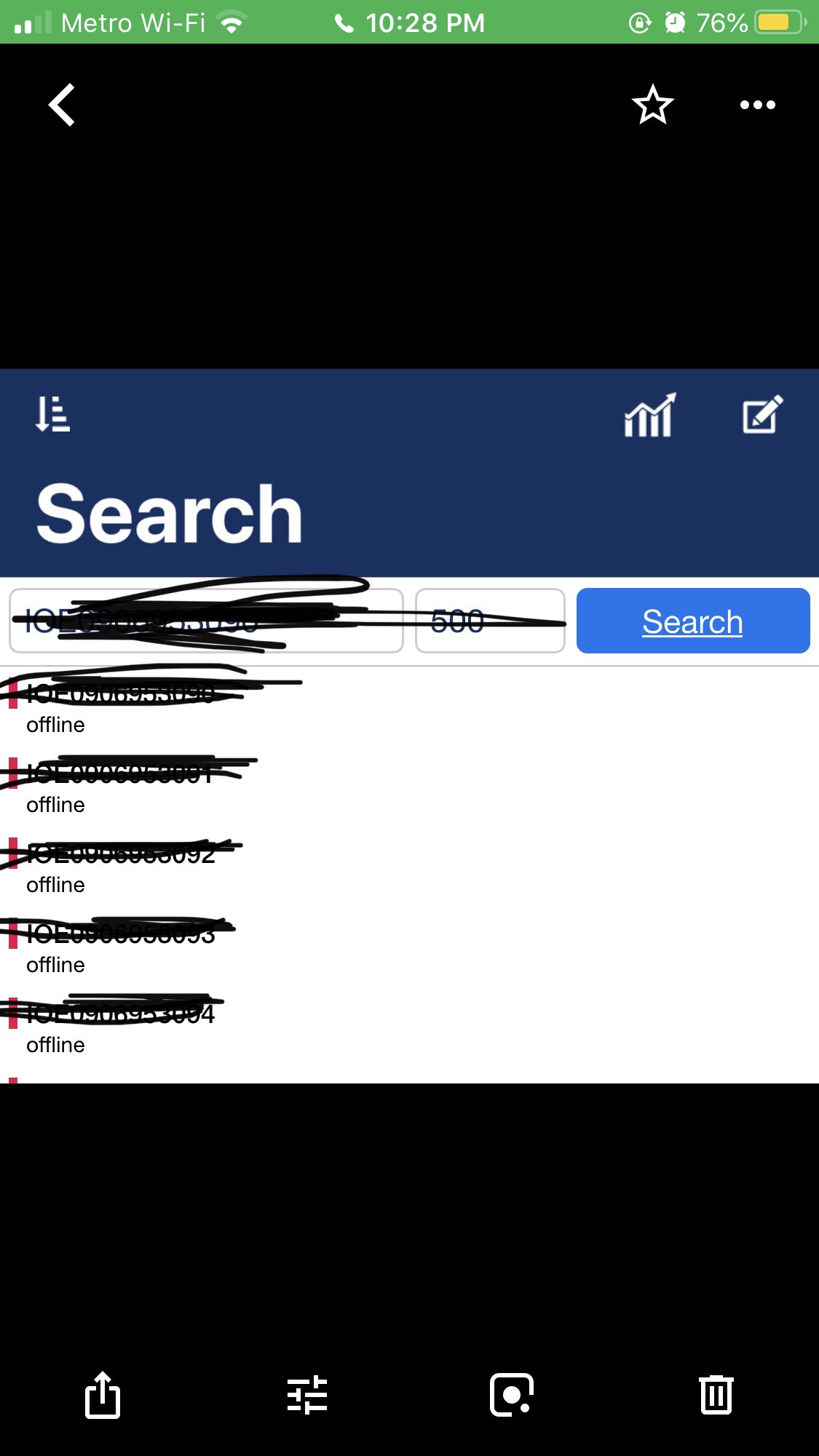A detailed image caption for the described screenshot:

The image captures a meta-screenshot (a screenshot of a screenshot) displayed on an iOS device, exhibiting the phone's status bar, app interface, and multiple layers of content. At the very top, the status bar is highlighted in green, indicating an ongoing call. From left to right, a two-bar cellular network icon displays the carrier "Metro," followed by a Wi-Fi icon and a time stamp reading "10:28 PM." Next to the time, a call icon is visible, suggesting an active call. The right side of the status bar includes an orientation lock icon, an alarm icon, the text "70%" indicating the battery percentage, and a yellow battery icon.

Below the status bar, a black header houses a white back arrow on the left and two icons to the right: a star and a three-dots menu. Dominating the central portion of the screen is the main screenshot, which appears to be the results of a search query. The top portion of this embedded screenshot features a prominent blue bar containing a sort icon, a second sort icon, and an arrow pointing to the right. Below this bar, "Search" is bolded in white text. The search box beneath shows black scribbles obscuring the original search term, a "500" number beside it in a secondary search box, and a blue button labeled "Search."

The search results, which are also scribbled out with black markings, occupy the space below the search box. Each result is marked with an "offline" label on a white background. At the bottom of the main screenshot, another black space spans the width of the screen, above a set of buttons aligned in white: an export icon, a settings icon, a lens icon, and a delete icon. This intricately layered capture highlights the use of the iOS photo app in managing screenshots and search results.